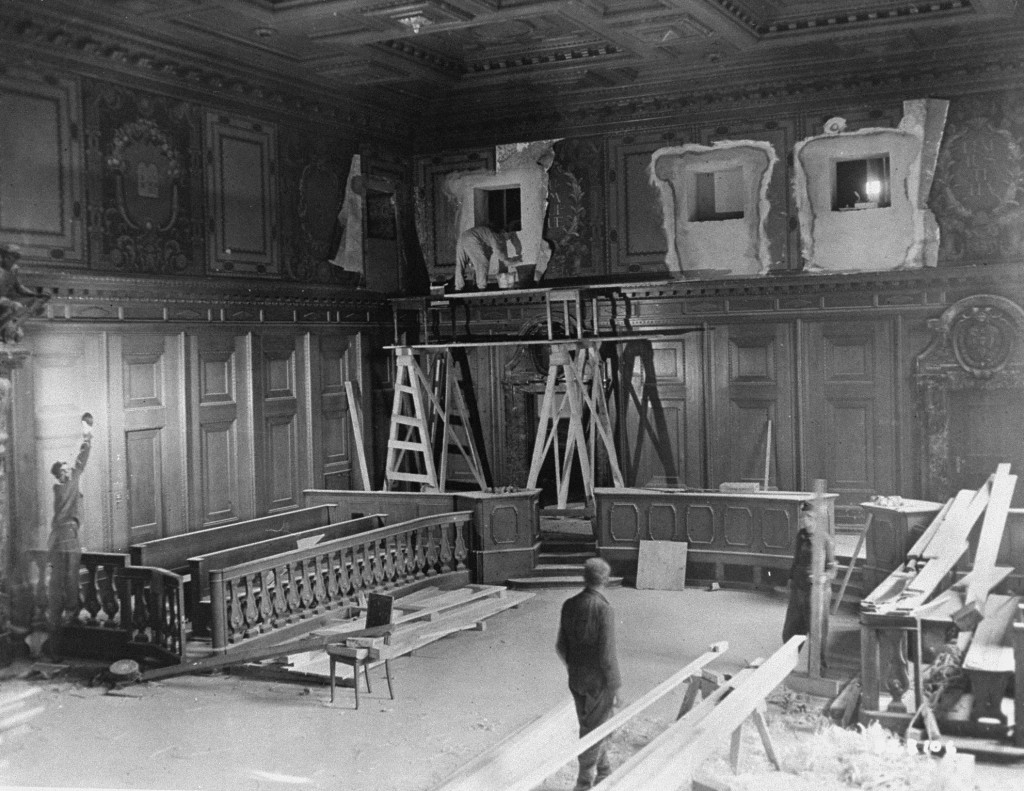This black-and-white photograph, likely from the early 20th century or earlier, captures the detailed interior of what appears to be a courtroom undergoing renovation. The spacious room features high, ornately decorated wooden walls adorned with shaker-style craftsmanship and intricate ceiling designs composed of various squares and depths. The image is in landscape format and shows several rows of pews or benches on the left, suggesting accommodations for jurors.

Several workers are dispersed throughout the scene: one is high up on temporary scaffolding, attending to lighting and painting tasks near the ceiling. Another worker on the left appears to be painting or staining a section of the wall. In the middle ground, a man is walking past wooden planks supported on sawhorses, moving towards another man who stands about 10 feet away, holding a vertical board and watching the approach. The photograph is filled with wooden beams, planks, and other construction materials scattered throughout, underscoring the active refurbishing process in this intricately designed, multi-level space.